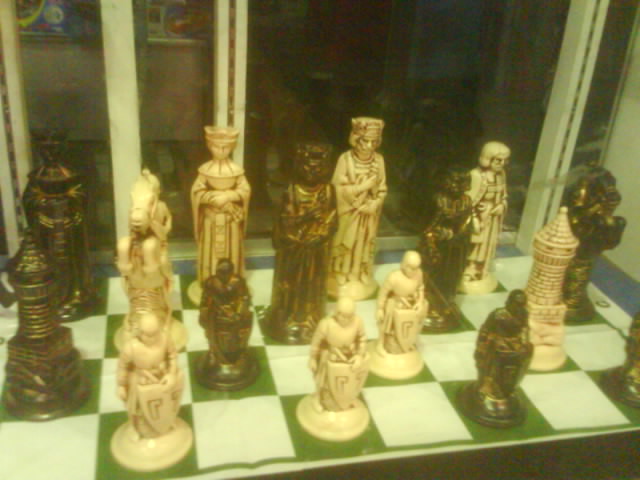This vivid display showcases a collection of intricately carved, ornate chess pieces set against a green and white checkerboard pattern. The checkered board appears to be a folded piece of fabric. The pieces themselves, which appear to be antique and crafted from materials resembling ivory and bronze, exhibit fine detailing. The pawns, clad in shields and armor, are lined up in the front, while the taller and more elaborate statues of the king and queen, complete with crowns and robes, dominate the back row. Knights are depicted as horse sculptures with riders atop. This display is housed within a glass case, with an obscured view through the window behind it, offering just a shadowy glimpse of a wall and darker background. The meticulous craftsmanship suggests each piece, whether an off-white or dark bronze color, holds historical significance and artistic value.